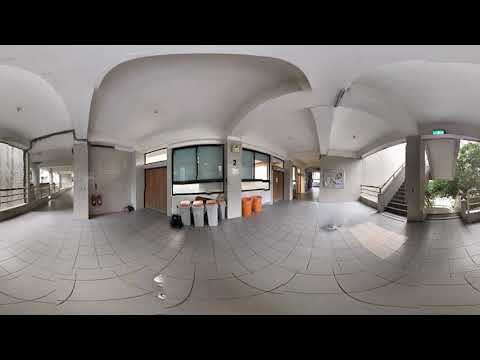The image depicts a fish-eye view of a roofed courtyard or patio, likely belonging to a residential building or hotel. The space features a floor made of gray stone tiles and white stucco or cement walls. The left side of the image reveals a window at the edge, leading to a well-lit hallway. In the center, directly in front of the viewer, there are two curved windows separated by a pillar, with several trash cans positioned below them, including three white and two orange ones. To the left of these windows, there is a wooden door. The right side of the image includes an outdoor, zigzagging staircase, with small trees or shrubs nearby. Additionally, there are doorways visible down a hallway on this side. The curved concrete ceiling adds to the enclosed, sheltered feeling of the space, while the presence of greenery and natural light from outside suggests a welcoming ambiance.